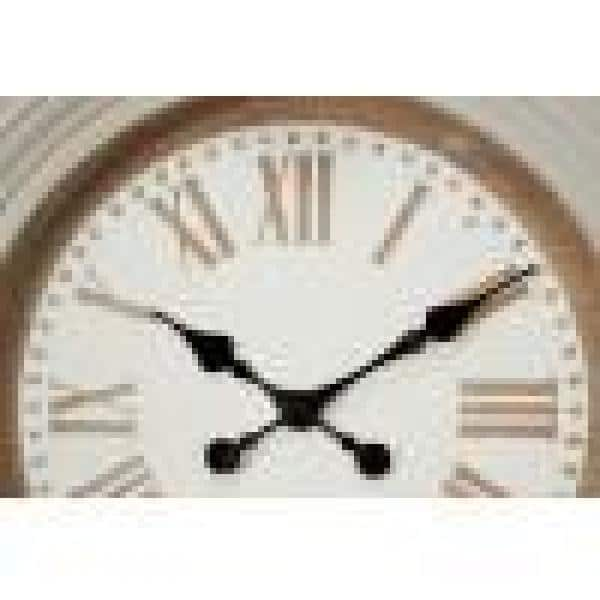The image depicts a highly pixelated, rectangular photograph of a wall clock, with noticeable details despite the blur. The clock features a circular face with a light brown, wooden-esque border and displays Roman numerals instead of numbers. The clock's white face includes tan-colored notches and distinctive black hands—the hour and minute hands both pointing towards the 10:10 position. The hands have ornate designs: long points on the minute hand and hour hand with spade-shaped ends, while the opposite ends have round circles. The clock's outer edge has a layered, 3D appearance, painted white to enhance its intricate look. Notably, the bottom portion of the clock, including the numerals VI (6) to X (10), is cut off and out of the visible frame.